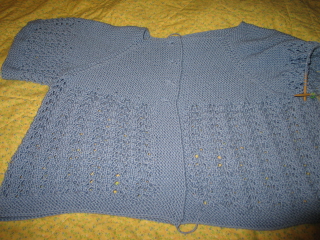This square color photograph features a light blue knitted women's blouse with short sleeves, neatly draped on what appears to be a polished wooden surface partially covered by a yellow bedspread. The blouse is buttoned down the center with four visible buttons, running from the neck to the hem. A small loop of loose thread is evident at the bottom of the blouse. The visible right sleeve and lower part of the blouse showcase a brocade or embroidered design, adding a subtle texture to the fabric. The photo does not contain any other objects or elements, focusing entirely on the neatly displayed garment.